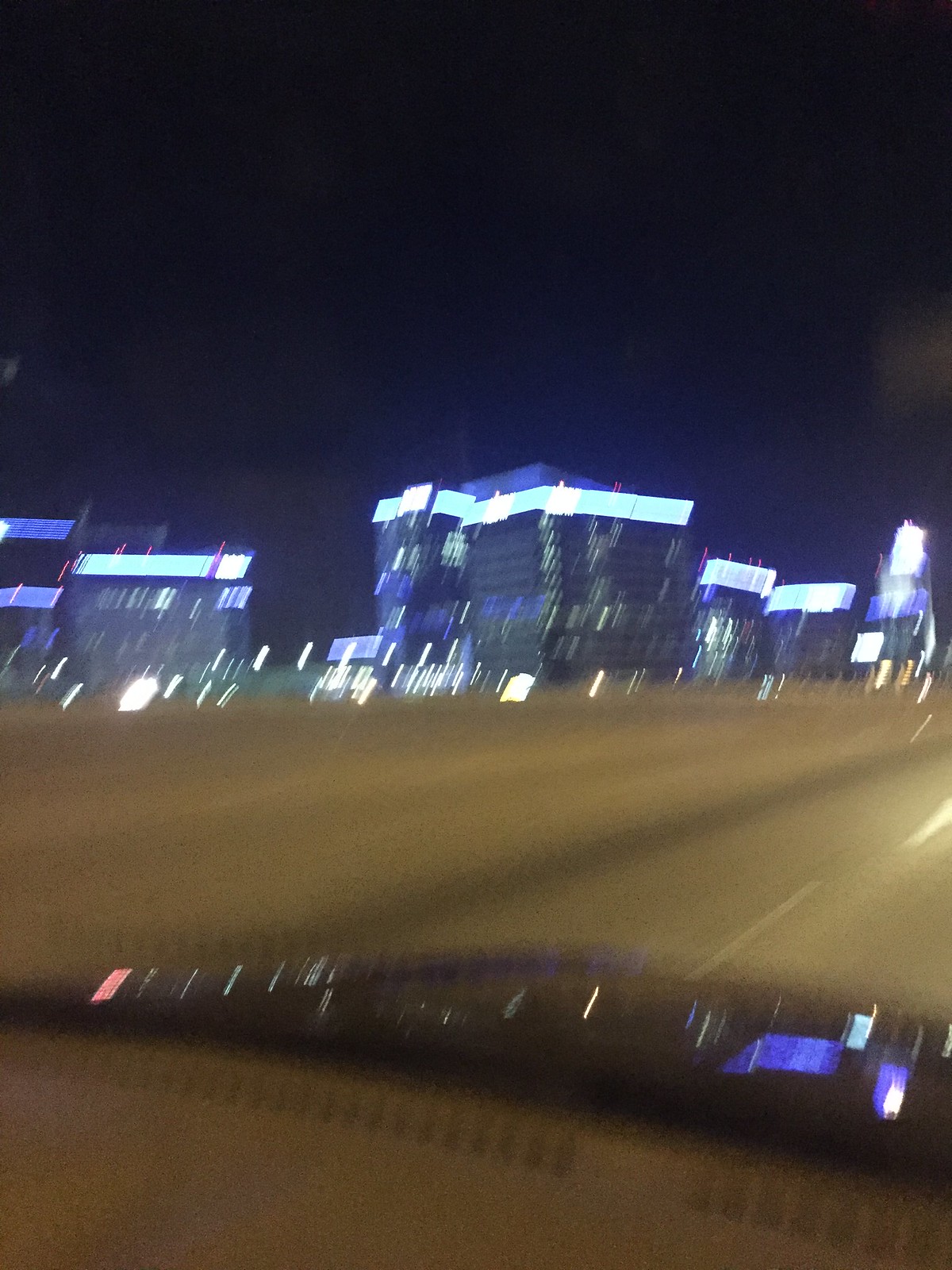A highly blurry nighttime photograph or artwork capturing a cityscape. The central focus is several large, illuminated skyscrapers that are visible but heavily obscured by the image's lack of clarity. The buildings are set against a dark blue sky, with potential reflections or lights making the scene seem even more abstract. The lower portion of the image depicts a wide street, tinged brown, suggesting the photo is taken from the opposite side of this road. The overall composition is ambiguous, with the blurriness creating streaks and lending an almost painterly quality, making it difficult to determine if the image is a photograph or an artistic rendering.